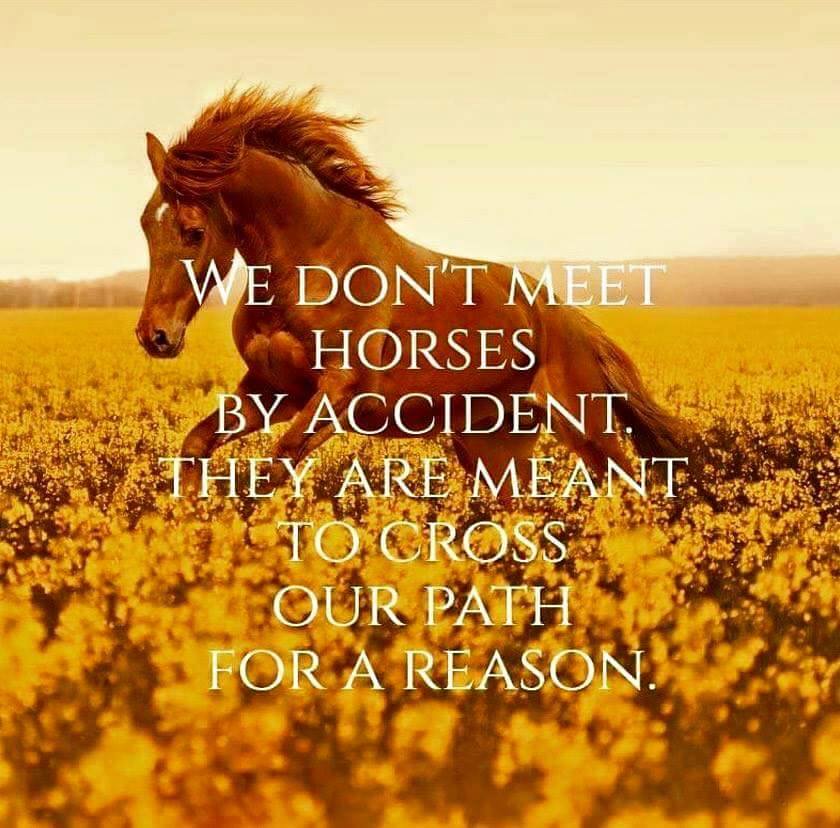The image shows a serene meadow with golden flowers, dominated by a majestic, reddish-brown horse galloping through the field from right to left. The horse, featuring a distinctive white star on its forehead, is captured mid-stride with its mane flowing, exuding grace and freedom. The scene is set against a distant backdrop of gentle brown mountains, stretching horizontally across the horizon, and a pale gold sky above. The lower two-thirds of the image is filled with the vibrant meadow, while the upper third consists of the tranquil sky and mountains. Superimposed in bold white, all-caps text is the inspirational quote: "WE DON'T MEET HORSES BY ACCIDENT. THEY ARE MEANT TO CROSS OUR PATHS FOR A REASON." This striking blend of photographic realism and graphic typography makes the image reminiscent of an inspirational poster or social media post, particularly appealing to horse enthusiasts.